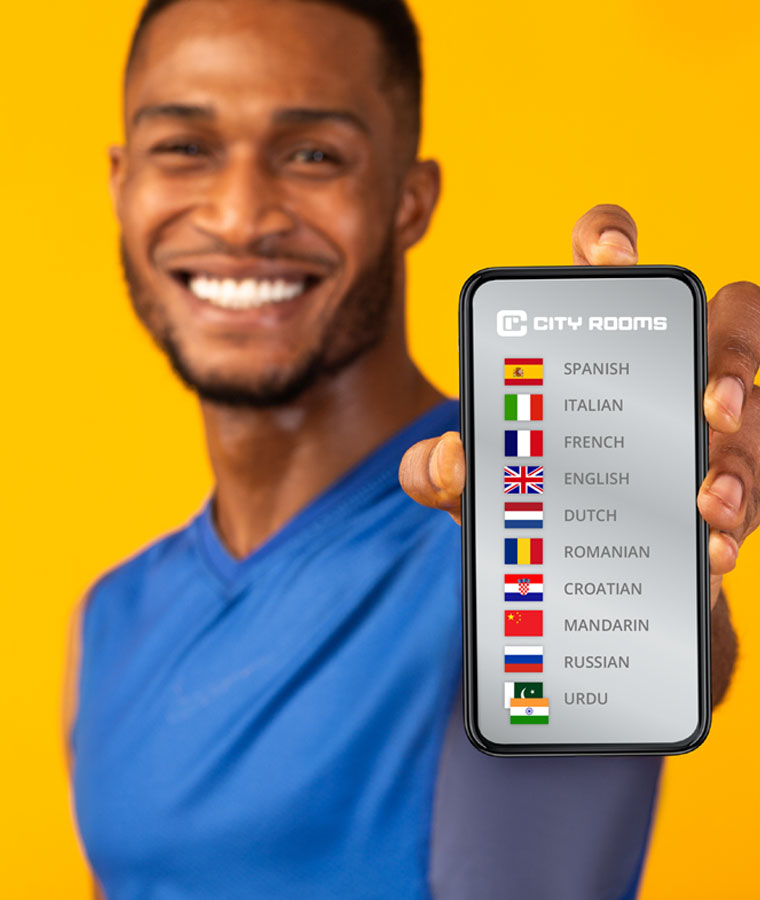A vibrant and eye-catching advertisement likely designed for a website features a digitally rendered image of a cheerful Black man. He appears to be around 35 years old, sporting a short, scruffy beard and a meticulously groomed razor line along his scalp. His smile is bright and inviting, showcasing perfect teeth, and his eyes reflect the same joyful energy.

He is dressed in a light blue, semi-shiny, short-sleeved synthetic shirt that resembles a soccer jersey, though it lacks any logos or printing. His left hand, in sharp focus, extends toward the camera, holding a smartphone prominently displaying an interface.

The phone screen showcases a mock-up application named "City Rooms," with the app's logo characterized by a large "C" encompassing an inserted "R." Below the logo, an array of flags representing various countries and languages, including Spanish, Italian, French, English, Dutch, Romanian, Croatian, Mandarin, Russian, and Urdu, suggests the app offers multiple language options, likely for communication or language learning purposes.

The background is a bright, attention-grabbing yellow, enhancing the overall high-contrast and upbeat aesthetic of the advertisement. Notably absent are any website details or additional context, further indicating that this image might be a mock-up or a composite of several different visual elements.